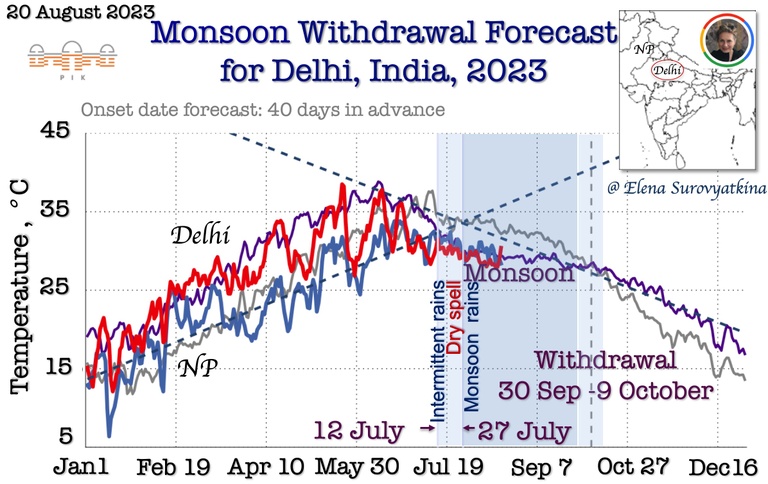This image depicts a detailed weather chart titled "Monsoon Withdrawal Forecast for Delhi, India, 2023," prominently shown at the top. In the top left corner, the caption mentions "20 August 2023" with a logo beneath it, and on the top right, there’s a small map indicating Delhi's location in India. The chart integrates a line graph tracking temperatures from 5 to 45 degrees Celsius on the left axis and dates ranging from January 1st to December 16th along the bottom. The line graph features blue, purple, and red lines representing temperature changes across these dates. The graph also identifies specific periods, such as the monsoon withdrawal between September 30th and October 9th, where a noticeable decline in temperature is observed.

Additionally, the chart overlays information about the monsoon activity, indicating phases of intermittent rains, dry spells, and significant monsoon rain periods. Annotations enrich the graph by noting the onset date forecasted 40 days in advance and a copyright attribution to Elena Suryakina. This comprehensive chart serves to illustrate the fluctuations in temperature alongside critical monsoon events throughout the year.